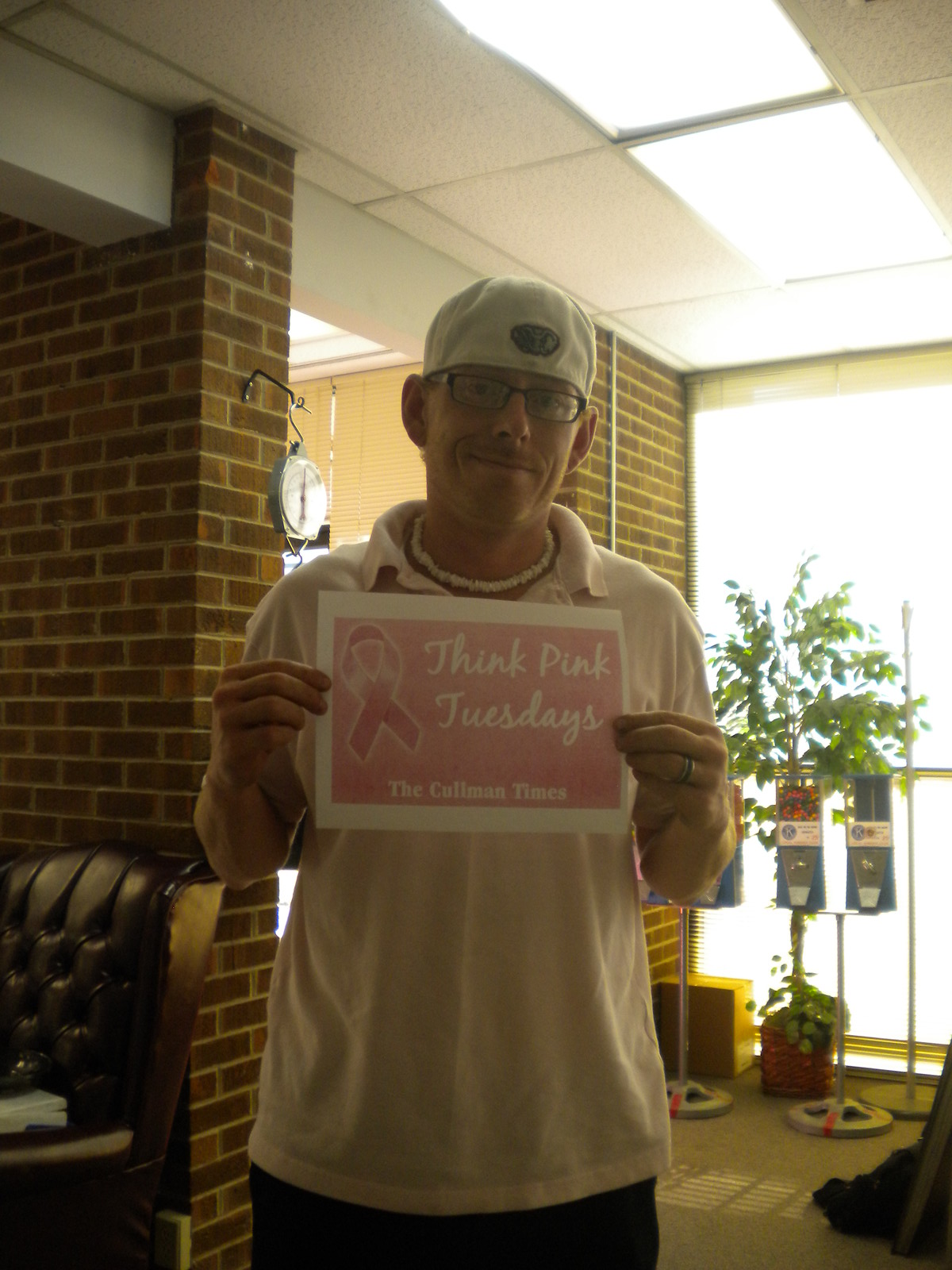In this daytime, full-color photograph, a man is prominently positioned at the center of a brick-walled room that could be an office, potentially administrative or educational. He is wearing a backwards white baseball cap, dark-framed glasses with clear lenses, and a necklace of white seashells. His attire includes a collared shirt that appears white in some descriptions, though possibly pink. He is holding a standard letter-sized sign with a white border and pink interior, featuring the text "Think Pink Tuesdays" in a cute cursive font. A pink ribbon, symbolizing breast cancer awareness, is placed to the left of the text, accompanied by the tagline "The Kauffman Times" at the bottom. Surrounding elements of the room include a black leather chair to his left, candy dispensers behind him to the right, and a fake tree in front of a large window that allows daylight to flood the space. A couple of overhead lights provide additional illumination.